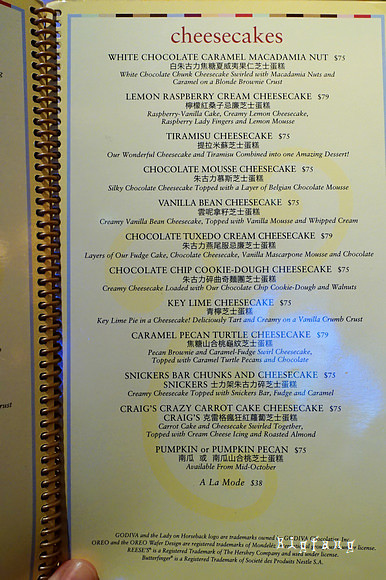An open menu book is displayed, showcasing the cheesecake section. The menu is bound with a spiral spine, reminiscent of a high school notebook, visible along the inner edge. The left page features a distinct yellow border that encloses a secondary blue border, which frames a narrow strip of the white content area where the food information begins. The right page is fully visible, bordered by yellow along the top and left edges, with an interchanging pattern of white, blue, and brown across the top edge.

Dominating the top center of the right page, the word “Cheesecakes” is prominently printed in large red letters. Below this header, written in black, is the title “White Chocolate Caramel Macadamia Nut,” followed by the price, which is partially obscured. This description is accompanied by information presented in both Chinese and English. The menu lists an additional 11 desserts, each with the dessert name and corresponding price on the right side, followed by brief descriptions in Chinese and then English beneath each entry. A thumbnail peeks in just to the right of the spine at the bottom of the right page, likely positioned to turn the page.